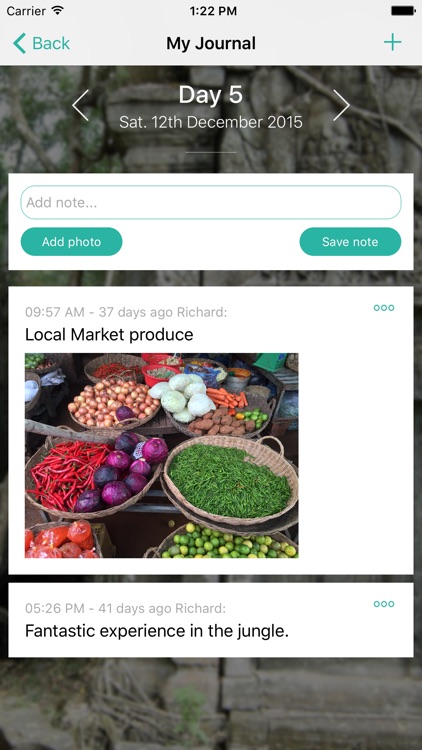The screenshot shows an overview of my experience using the "My Journal" app on my phone, featuring Day 5, Saturday, December 12, 2015. The interface allows me to add and save notes in a teal blue color or attach photos using a teal blue button. Notably, at 9:57 AM, 37 days ago, Richard sent a picture of local market produce, which appears as a message. Another message from Richard, sent at 5:26 PM, 41 days ago, describes a fantastic experience in the jungle. The app displays my phone's screensaver in the background, and each message is accompanied by three small buttons for additional actions, such as confirming receipt or dismissing the message.